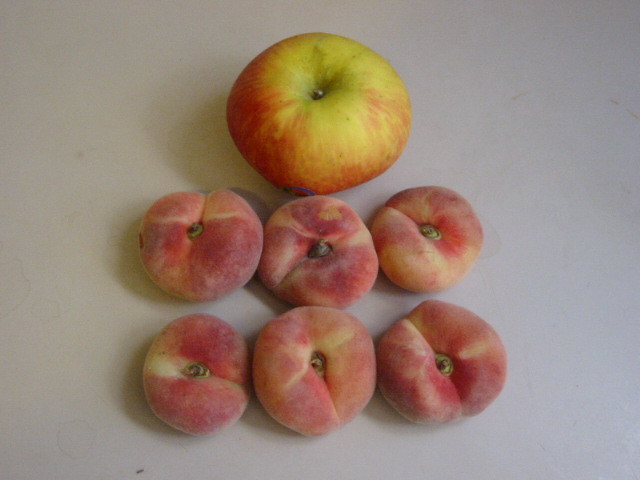The image depicts a meticulously arranged assortment of fruit on a light orchid-colored backdrop. At the top of the display is a single apple featuring a gradient of colors: a greenish-yellow at the top near the stem that blends into a deep red on the sides. The apple, which has a round, blue sticker with red and black print, stands alone above two neat rows of small peaches—three in each row. The peaches, significantly smaller than the apple, exhibit a captivating combination of deep reddish-purple hues interspersed with lighter yellow tones and faint white lines. Each peach has a tiny stem, adding a touch of authenticity to their fresh appearance. The overall composition, set against a soft background, highlights both the vivid colors and the meticulous arrangement of the fruit, making them appear particularly appealing.